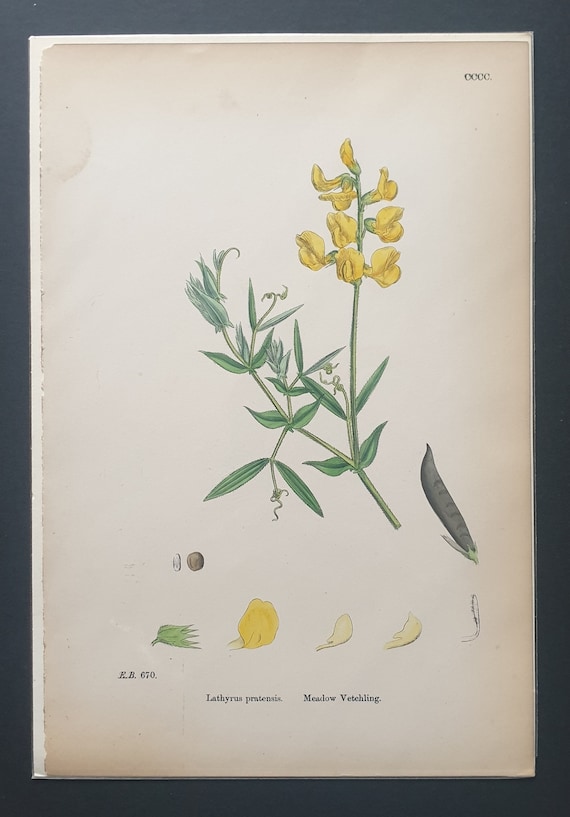The image is a detailed depiction of botanical art, seemingly a photograph of a historical illustration. The artwork is presented on a piece of aged, beige parchment paper mounted inside a one-inch black picture frame, against a dark bluish-gray background. The central focus is a drawing of a Meadow Vetchling (Lathyrus pratensis). The illustration shows a stem that splits into two directions: the right side showcases multiple small yellow flowers blooming along the upward stretch, each flower delicate and pointy. At the very tip, another yellow flower blooms prominently. The left branch displays various green leaves, ending in a small cluster of three or four leaves. Additionally, a darker rendition of a peapod appears towards the middle right of the image. Below the main plant illustration, there are detailed diagram sections outlining different developmental stages and parts of the plant, including individual petals and leaves. The top right corner of the page is marked with "CCC," while the bottom bears the identifier "EB670" alongside the handwritten text, "Lathyrus pratensis, Meadow Vetchling."